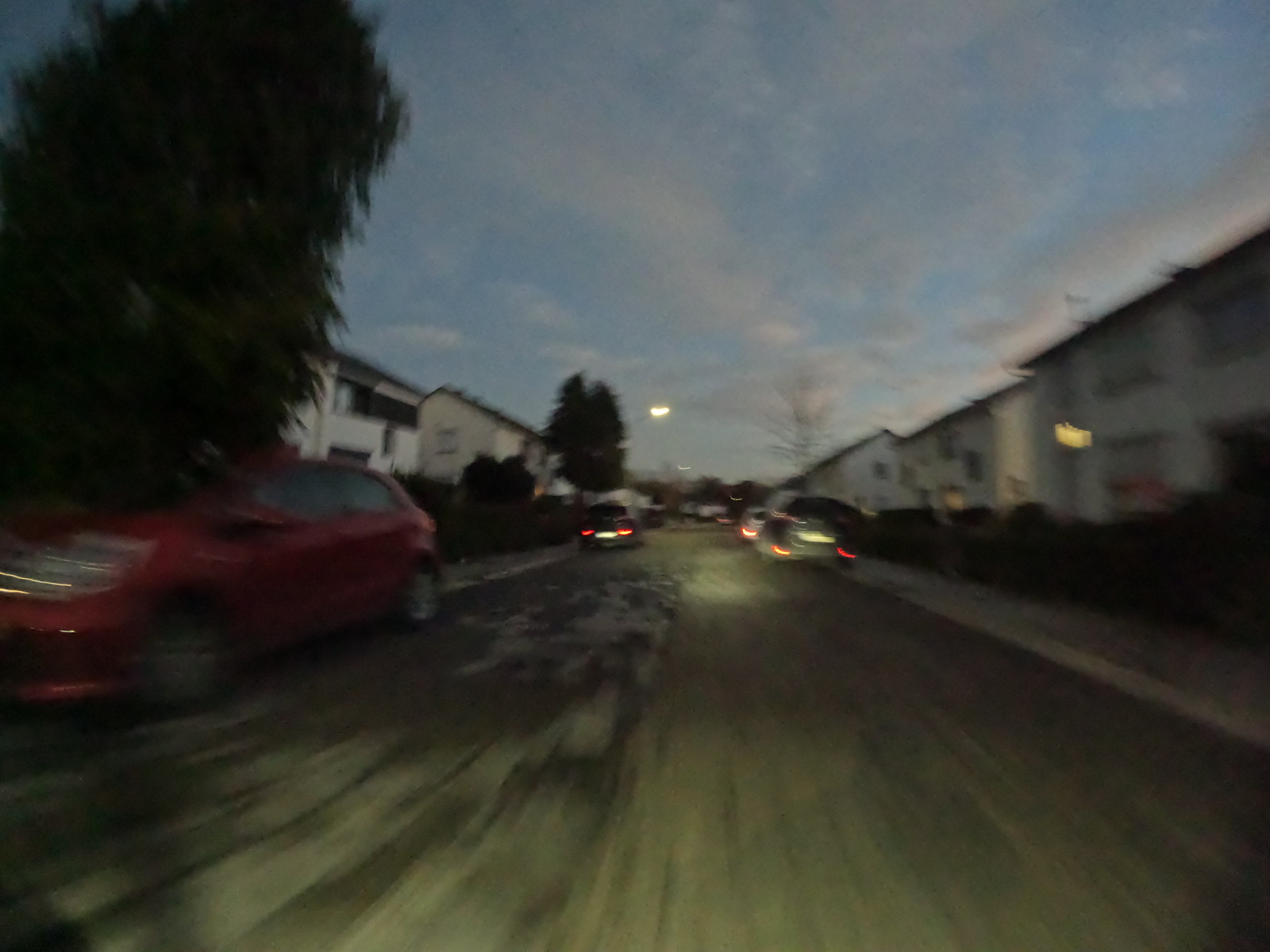A blurry photograph, likely captured by a dash cam positioned at the front of a car, depicts a concrete road with various vehicles on either side, some of which appear to be parked. The scene suggests movement, perhaps as we travel down the road. White, two-story houses line both sides of the street. Taken during the early morning or late evening, the dim lighting and active headlights of the vehicle from which the image was captured indicate a time around sunrise or sunset. The sky overhead is mostly cloudy with blue hues, enhanced by the soft tints of the dawn or dusk. On the left side of the road, we are approaching a red, four-door car, facing us, which adds a sense of direction and depth to the image. The overall atmosphere is serene and somewhat introspective, conveyed through the subdued lighting and the everyday scenery.